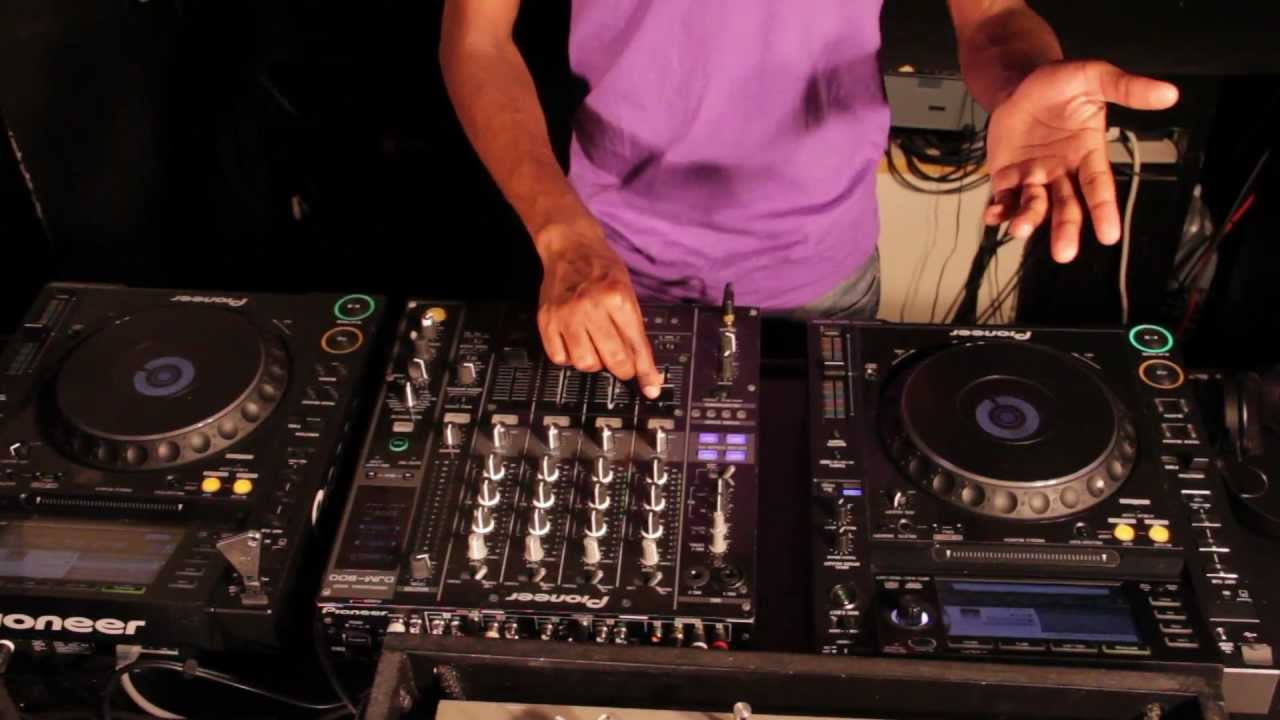In a dimly lit room, a DJ is intently working a turntable, partially shown from the torso down. The DJ is donned in a mostly purple shirt, branded with "Pioneer" on the turntable. He is maneuvering controls on the DJ board: his right hand adjusts a lever while his left hand hovers with fingers splayed, perhaps moving with the rhythm. The DJ board brims with gray knobs and white switches. Flanking the board are two round speakers with metallic rims and purple centers, each ornamented with tiny circlets, with illuminated green and orange circles behind them. A white wire dangles near the DJ's right hand, adding to the scene’s intricate setup of technology and color.